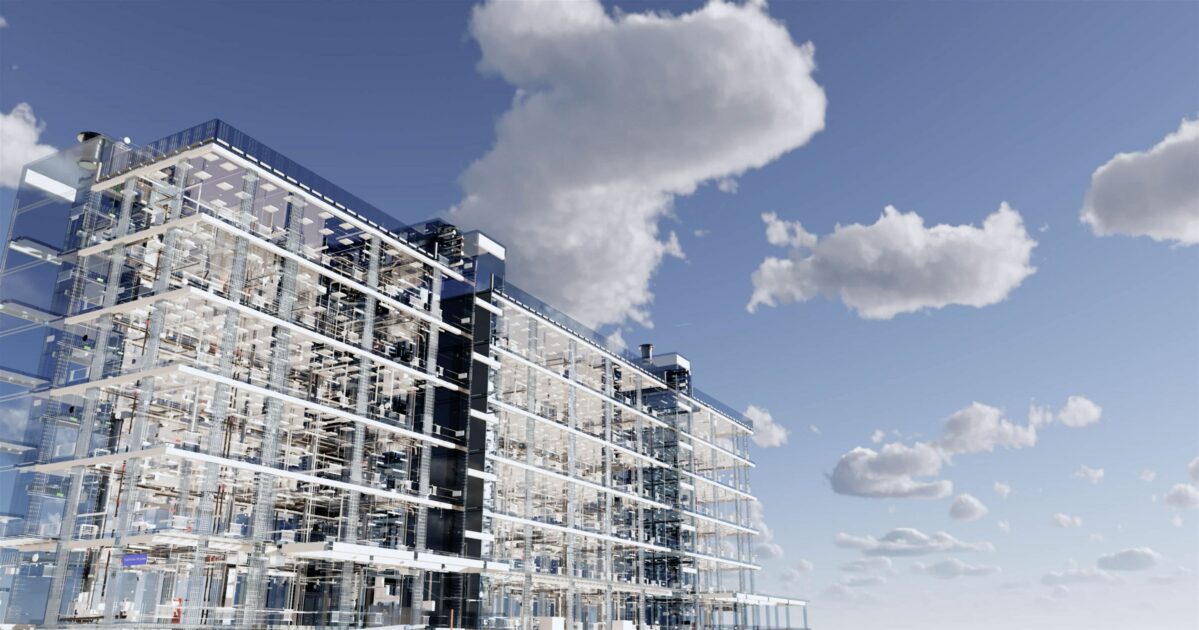The image depicts a tall, modern skyscraper, primarily constructed from clear glass that gives it a see-through appearance. The building is divided into three distinct vertical sections by two darker, black lines, likely housing elevator shafts. This segmenting adds to the sleek, futuristic look of the structure. The skyscraper, depicted from an angled perspective, occupies the lower left side of the image and extends downwards towards the right, aligning with the 10 or 11 o’clock position on a clock face. Only six floors of the skyscraper are visible, each well-lit, emphasizing the bright interior lights and the reflective, silvery-white exterior. The top of the building is outlined in a dark blue shade, contrasting with the predominant whites, grays, and blacks of the building. The background transitions from a dark to light blue sky, adorned with big, fluffy white clouds predominantly scattered on the right side, enhancing the overall vividness and clarity of the outdoor scene.